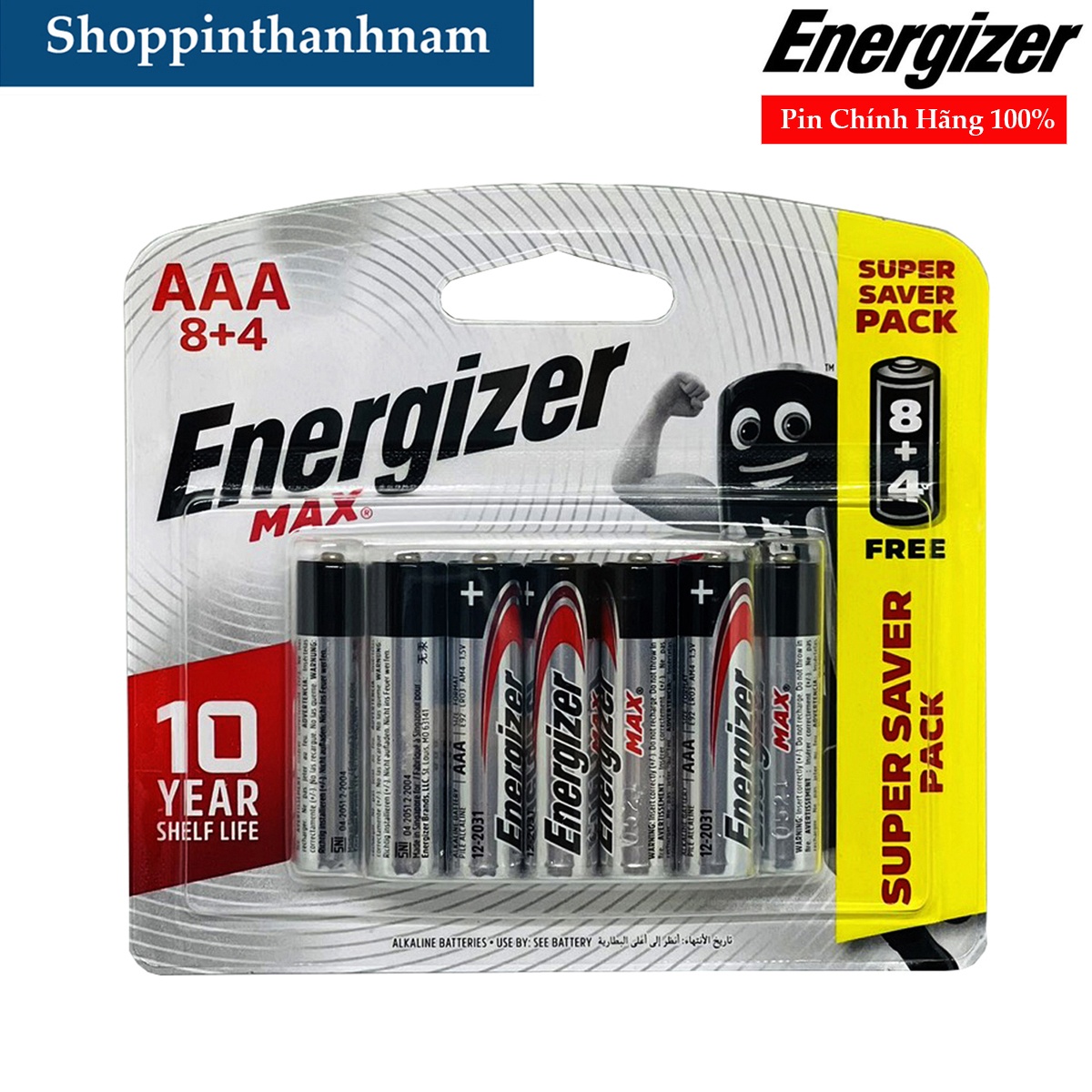In this detailed image, the focus is on an Energizer battery pack prominently featuring the Energizer logo on the top right corner, accompanied by the phrase "Pinching Hang 100%". To the top left, the text "Shopping Dan Ham" is visible. The pack contains a total of 12 AAA batteries, organized in a clear blister packaging. The packaging is labeled as a "Super Saver Pack", highlighting an "8 plus 4 free" offer. Additionally, the pack boasts a "10 years shelf life" guarantee from Energizer. The dominant colors in this image are yellow, red, black, and white, creating a vibrant and eye-catching presentation. There are no other notable details in the image.